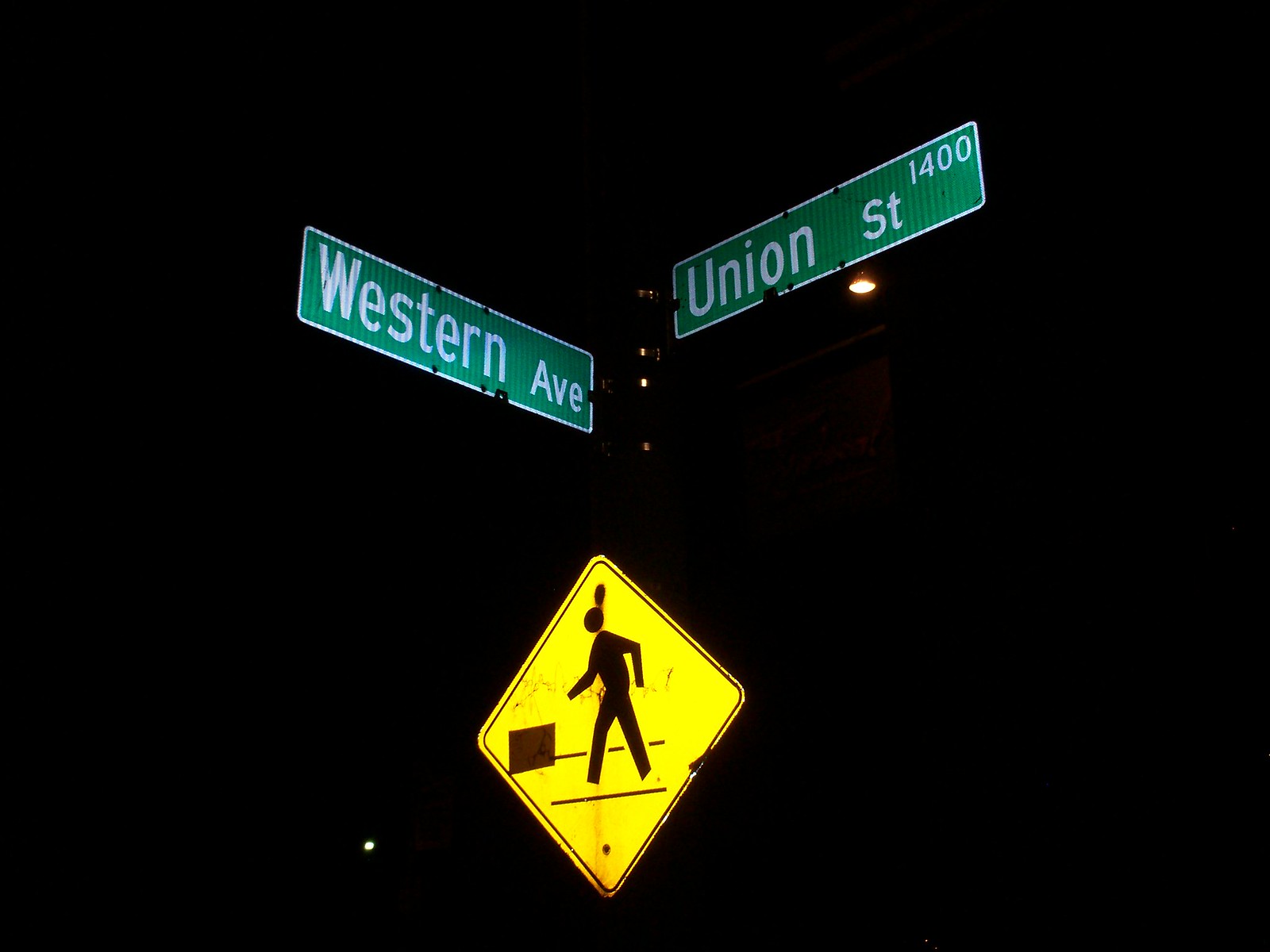In this nighttime image, a dark, almost pitch-black background contrasts starkly with the illuminated objects in the foreground. Dominating the scene are two green, rectangular street signs mounted on a pole. The sign on the right, "Western Avenue," is labeled in bold white print. To its left, another green sign reads "Union Avenue 1400" in the same white print. Beneath this sign, a streetlight casts a bright glow, though the pole itself remains shrouded in darkness except for where the light hits.

Positioned a bit lower on the pole is a yellow, diamond-shaped caution sign with black trim, depicting the silhouette of a person walking across a street. Below this, there's a smaller, horizontal line, presumably indicating a crosswalk, and a black square situated in front of the walking figure's silhouette on the sign. The overall composition captures a vivid yet eerie snapshot of urban infrastructure, emphasized by the contrasting darkness and artificial lighting.